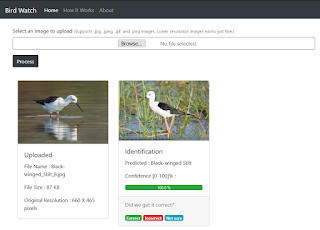This screenshot captures a compact website interface dedicated to bird watching. At the very top, there is a horizontal blue bar prominently displaying the title "Bird Watch." Directly beneath this bar is a sentence that is not legible in the screenshot. Below the sentence, there is a search box that allows users to browse the site, accompanied by a black button with white text.

Further down, there are two distinct photographs of birds. The first image features a black and white bird with horned legs, reflected beautifully in the water. The second image showcases the same bird standing amidst grassy, watery terrain. The term "identification" is partially visible in this section.

Towards the bottom, there is a horizontal green bar followed by a combination of green, red, and blue indicators with a caption that seems to inquire about the accuracy of certain information, presumably asking, "Did we get it right?"